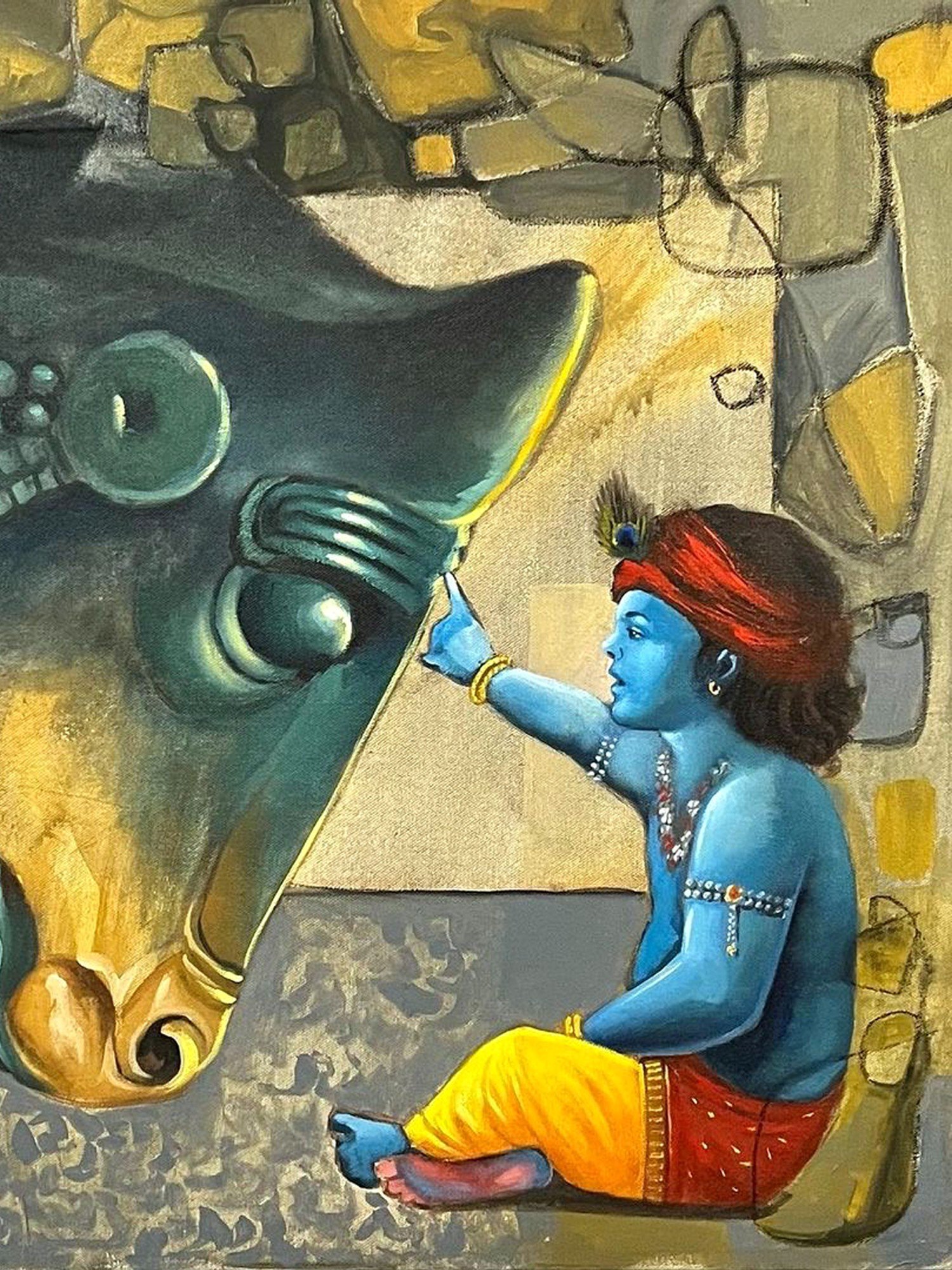This detailed painting depicts a young, blue-skinned figure, representing the Indian god Hare Krishna, dressed in yellow trousers and a red shirt while adorned with various forms of jewelry, including gold bracelets, a gold hoop earring, and a beaded necklace. A red fabric is wrapped around Hare Krishna's head, complemented by peacock feather-like decorations. Hare Krishna is seated, gently touching the bridge of a black horse's nose with his index finger. The horse, featuring a yellow nose, is solemnly bowing its head towards Hare Krishna in a gesture that indicates deep respect and a profound, intimate bond.

The background consists of an abstract array of yellow, grey, and black squares reminiscent of stone, with decorative elements that echo the colors of Hare Krishna's attire and the horse's nose. Additionally, there appears to be a subtle floral design within the background. The painting evokes a serene yet deeply spiritual interaction, encapsulating the reverence and mutual respect between Hare Krishna and the horse.